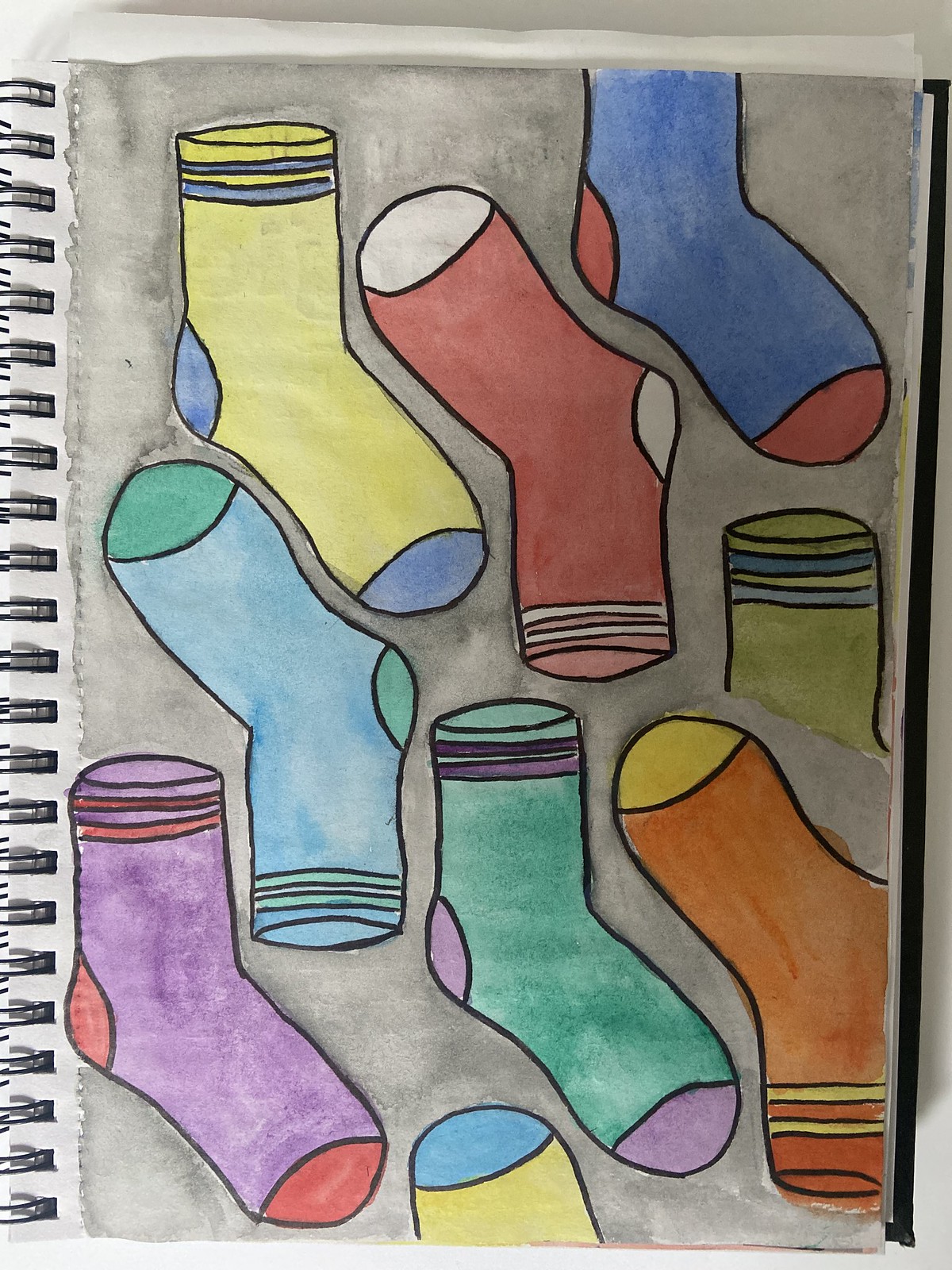This detailed watercolor and ink drawing is set on a gray background, filling a page within a spiral-bound sketchbook, with the silver wire binding visible on the left. The painting depicts nine colorful, illustrated crew socks, each with distinctive patches and stripes, all facing various directions. The socks include diverse and vibrant colors such as yellow, red, blue, orange, teal, and purple. Each sock features contrasting colors for the toes, heels, and stripes—such as a yellow sock with blue details, a red sock with white accents, a blue sock with red highlights, an orange sock with yellow features, and a green sock with purple embellishments. No text or words are present on the page.